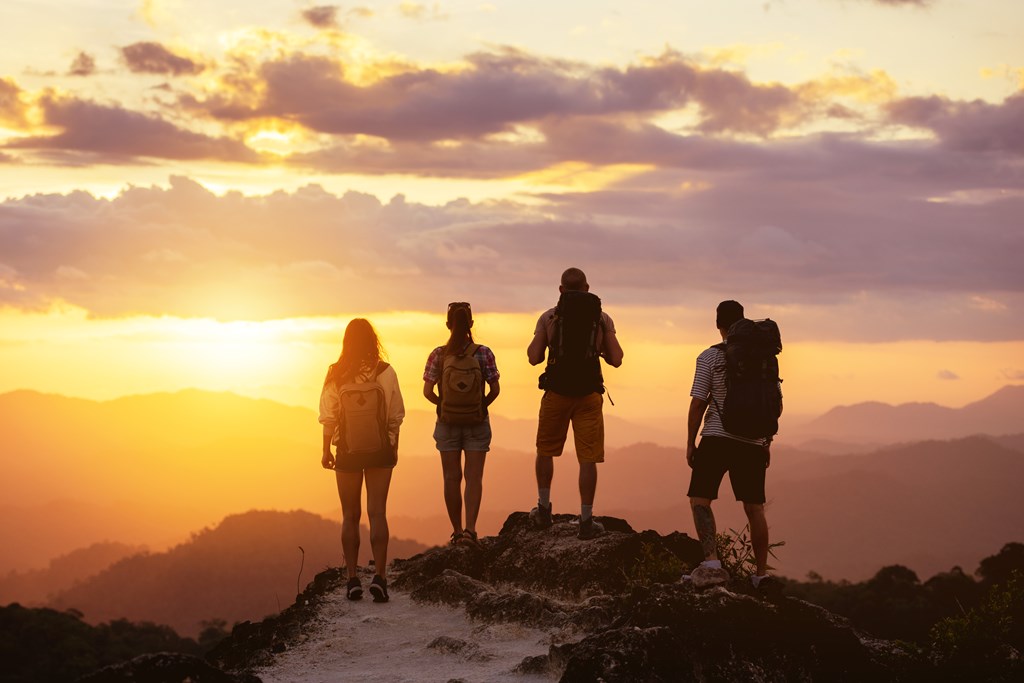The photograph captures four hikers—two women and two men—standing at the edge of a rocky mountaintop, gazing out over a valley framed by rolling hills and distant, bluish mountains. The hikers, dressed in shorts, hiking shoes, and backpacks, appear to be savoring the view after their climb. The scene suggests either sunrise or sunset, with a partly cloudy sky featuring dramatic, dark roll clouds and scattered purplish clouds. The atmosphere is rendered in delicate shades of orange and pink, with the sun low on the horizon. The women, one with brown hair and the other with red hair, stand on the left, while the two dark-haired men are positioned to their right. The hikers' backs are to the camera, creating a sense of shared accomplishment and serene contemplation amidst a panoramic, picturesque landscape.